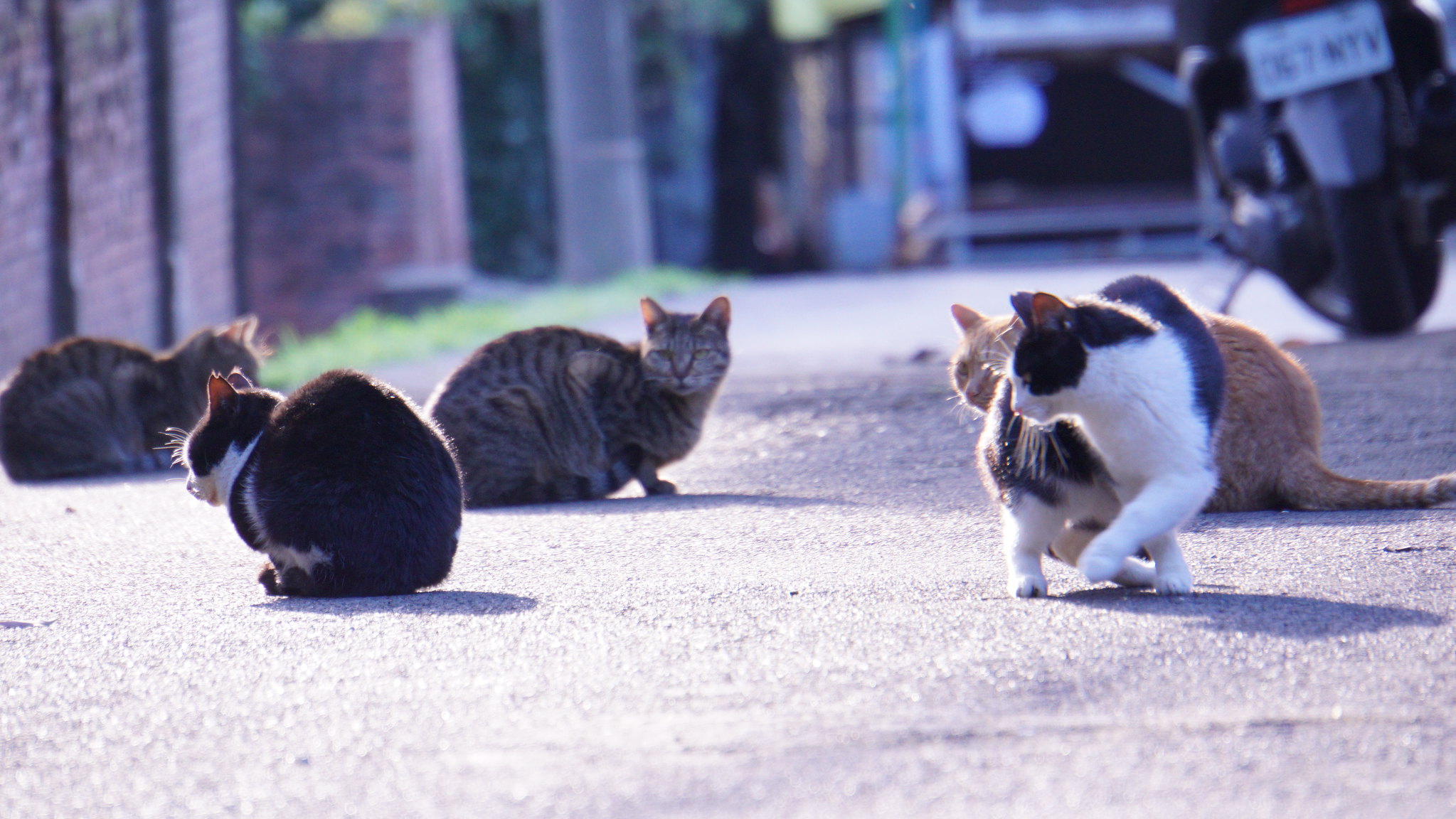In the bright daylight, five cats take center stage, sprawled across the grayish-black cement road. Two gray and black striped cats, relaxed and basking in the sun, lay to the left, while a mostly black cat with a few white spots sits nearby, looking to the left. Further right, an orange and white cat joins another black and white feline, but unlike its companions, this last cat stands as if stalking something unseen. The backdrop features a red brick wall to the left and the distant right reveals a sleek motorcycle with a white license plate that reads "067NYV." Beyond the motorcycle, there's a storefront adorned with a green sign next to a large glass window, framed by a short brown fence. None of the cats gaze directly into the camera; instead, they seem absorbed in their own world, under the bright sun.